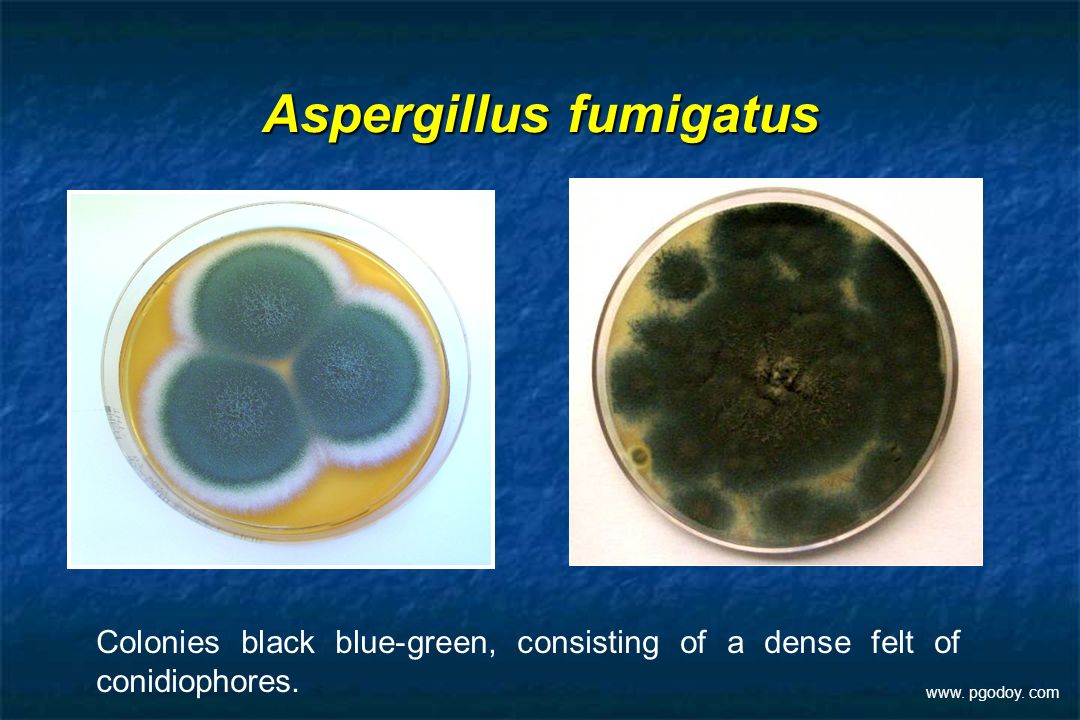The image displays a slide from a biology presentation. At the top, in yellow text, it reads "Aspergillus fumigatus." Below the title are two white squares positioned centrally, each containing a circular petri dish typically used in science labs. The dishes showcase different forms of the fungus Aspergillus fumigatus. The background of the slide is gradient, with dark blue at the top and bottom, transitioning to a medium textured blue in the middle, contributing to an aesthetically pleasing appearance.

The petri dish on the left contains three interconnected black circles outlined in white, set against a yellow liquid background, resembling the appearance of three eggs. The dish on the right displays a fuzzy, dark green and light brownish mixture, resembling algae found in a forest.

At the bottom of the image, white text provides additional context: "Colonies black, blue-green, consisting of a dense felt of conidiophores." In the lower right-hand corner, the website www.pgodoy.com is noted in small white letters.